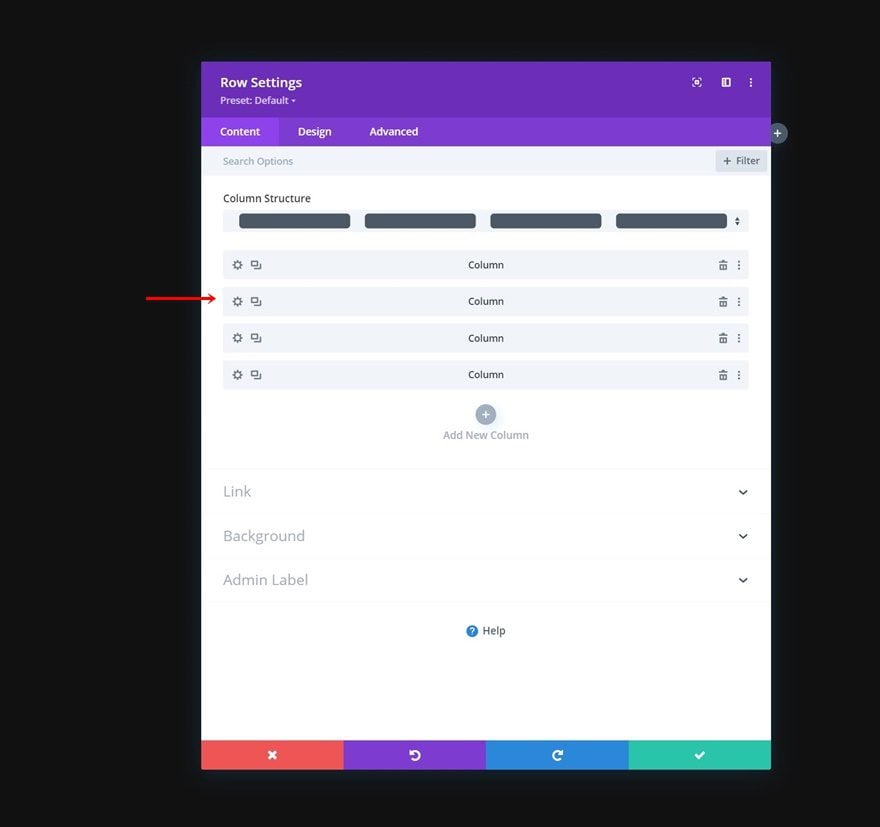The image showcases a configuration or settings interface with a predominantly black background. Centrally positioned is a detailed design interface with purple and white elements, transitioning into a colorful bottom section. At the top of the interface, the label "Row Settings" is prominently displayed, with the preset set to "Default." The interface is currently focused on the "Content" section, alongside tabs for "Design" and "Advanced" settings.

Within the "Content" section, several options are visible. The top portion includes a search bar and a filter button. Below that, a column structure is shown with four columns, highlighted by an arrow pointing to the second column, indicating a gear icon for additional settings. Adjacent to this, a plus button is provided for adding new columns.

Further down, there are specific sections for "Link," "Background," and "Admin Label," each with their own configurations. A small question mark icon labeled "Help" is also visible for additional assistance.

At the bottom of the page, there are four distinct buttons: a red button with an 'X' symbol for canceling, a purple button with a refresh icon for resetting changes, a blue forward button, and a green button with a check mark for confirming changes. This interface appears to be a detailed settings or customization menu, allowing users to modify content, design, and structure efficiently.